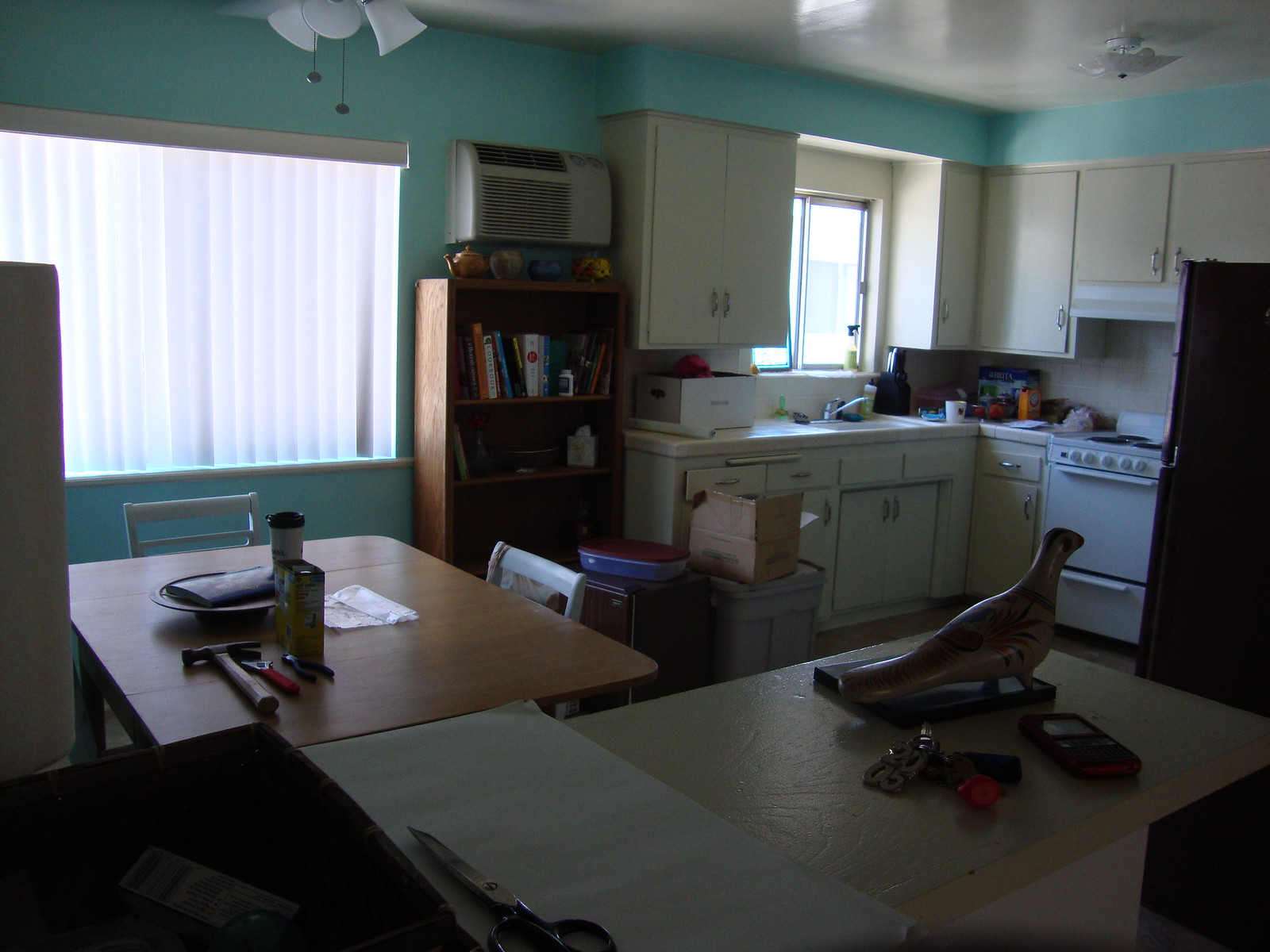A clean, well-illuminated kitchen is depicted in this full-view image. The left wall is painted in a greenish hue, complemented by a window dressed in white curtains. Light floods the scene from two ceiling-mounted lights: one positioned towards the left and another on the right, both emitting a soft white glow. The ceiling itself is a pristine white. Adjacent to the left window, a set of bookshelves is visible, housing numerous books and a variety of decorative items on top. Atop these shelves sits a unit that appears to be either a heater or an air conditioner.

On the right side of the image, an array of cupboards lines the wall, accompanied by a sink, stove, and refrigerator, creating a functional and organized workspace. Moving towards the foreground, two tables are cluttered with dishes, scissors, and various other items, indicative of recent activity. Two white chairs are positioned at these tables, seamlessly matching the overall light and airy aesthetic of the kitchen.